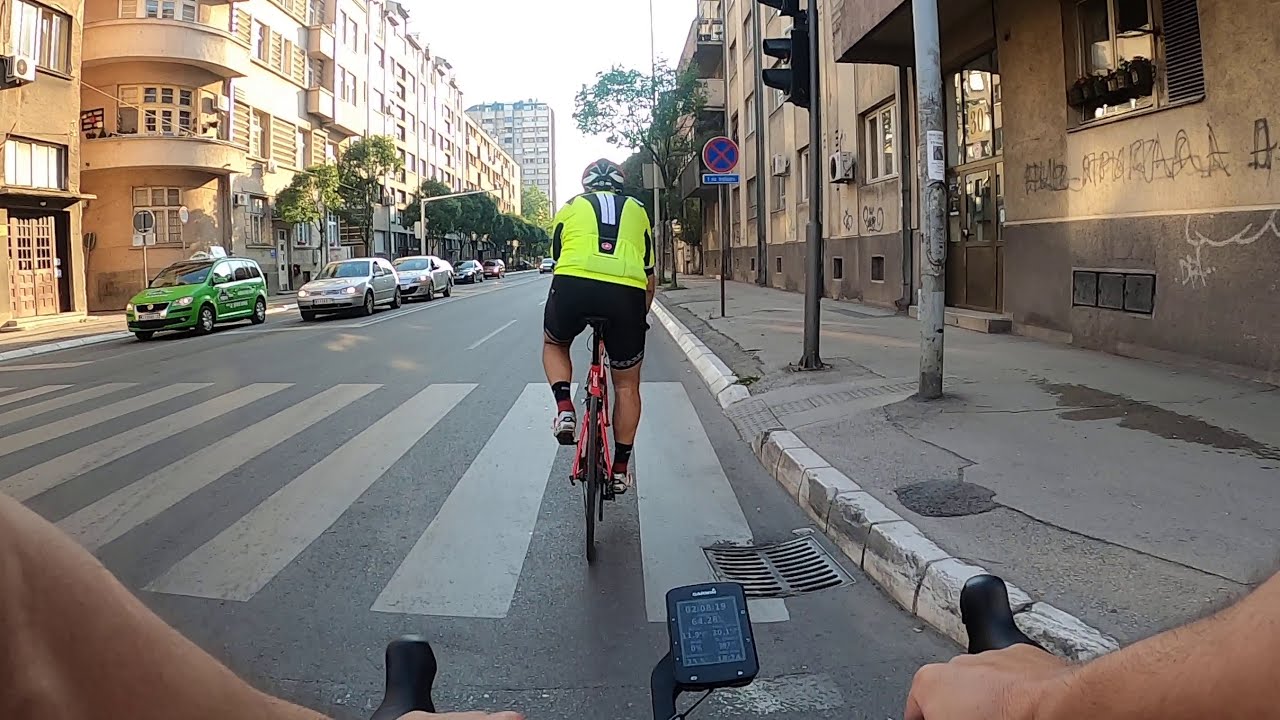This image captures the perspective of a bicyclist riding down an urban street, evidenced by their hands gripping the black handlebars at the bottom of the frame. In front of the rider is another cyclist on a red bicycle, dressed in black shorts and a fluorescent yellow short-sleeved top. This cyclist also wears white sneakers, dark socks, and a black-and-white helmet. Positioned slightly to the right near the curb, the cyclist's view includes several urban details: to the right is a series of various shades of brown and tan buildings, some appearing to be four to five stories high, featuring doors, windows, and graffiti-laden walls and poles. Along the patched-up sidewalk are scattered some green trees. On the left side of the street stand taller beige-brown buildings, also about four to five stories, interspersed with green leafy trees. Traffic flows on the opposite side of the road with several cars visible, including a green company car, two gray or white cars, a dark black car, and a reddish car, all seemingly halted. Prominently, a red X sign with blue elements and a blue placard below it are visible on the right. The scene is brightly lit, indicating it is daytime.